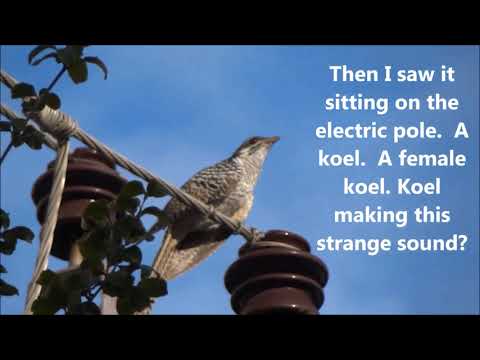In this image, a female koel, characterized by its tannish brown and gray feathers, is perched slightly off-center to the left on a tan piece of rope, which extends toward the left side of the picture. The bird's gaze is directed upwards at the blue, slightly cloudy sky that forms the background. Green leaves and branches from a nearby plant slightly obscure the electric pole she is perched on. Below the bird's feet, there is a brown object tied to the rope, mirrored by another identical object to the left of the bird. White text on the right side of the image reads, in sentence case, "Then I saw it sitting on the electric pole. A koel. A female koel. Koel making this strange sound?" Black banners frame both the top and bottom of the image.